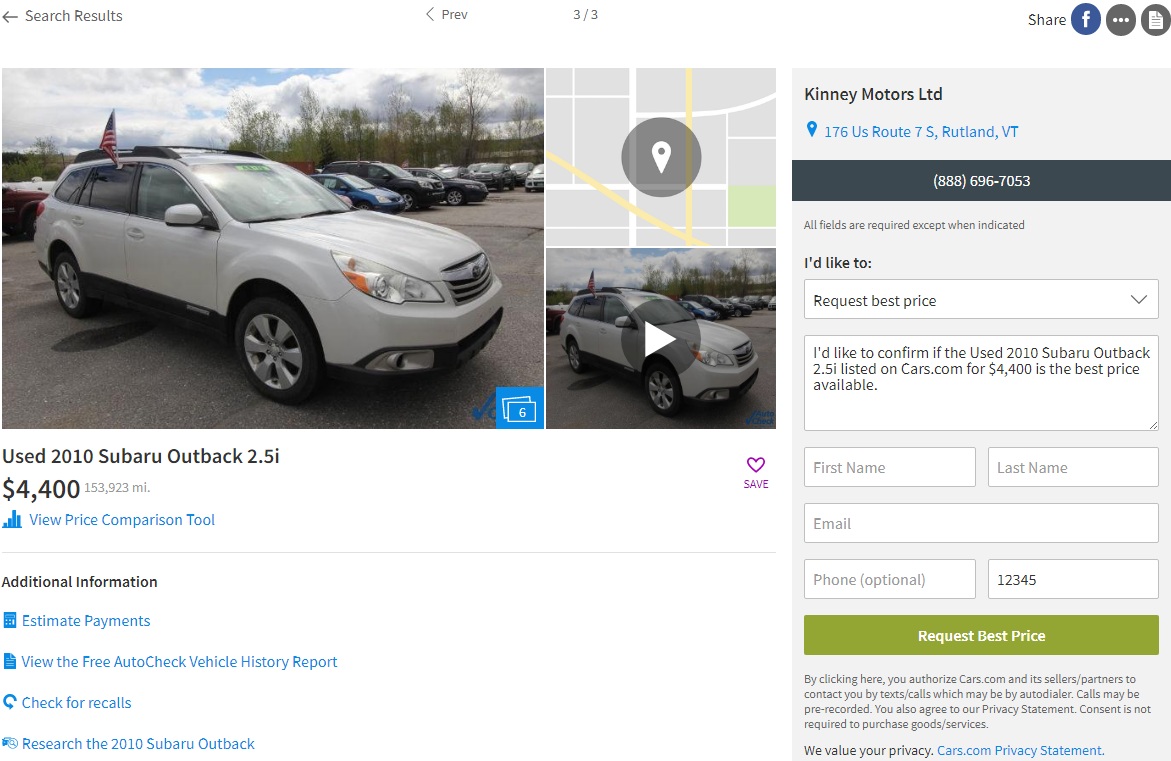Screenshot of Kenny Motors LTD website with a clean, white background. Positioned on the right-hand side of the page, the dealership name "Kenny Motors LTD" is prominently displayed. The location is specified as 176 US Route 7S, Rutland, Virginia. Directly below, a button allows users to initiate a call to the dealership at 888-696-7053. A notice below states "All fields are required except when indicated."

A form follows with a drop-down menu labeled "I'd like to," where the first option is "Request Best Price." The adjacent text box includes a preset message: "I'd like to confirm if the used 2010 Subaru Outback 2.5i listed on Cars.com for $4,400 is the best price available." Users are prompted to fill in fields for their first name, last name, email, phone number, and zip code. Completing the form, a "Request Best Price" button awaits submission.

On the left side, an image of a light gray used 2010 Subaru Outback 2.5i is prominently displayed, listed at $4,400 with 153,923 miles on the odometer. Below the image, options to "View Price Comparison Tool" and access additional sections such as "Estimate Payments," "View the Free AutoCheck Vehicle History Report," "Check for Recalls," and "Research the 2010 Subaru Outback" are available amidst a light gray divider line.

Adjacent to the car’s image, a small map with a pinned location shows exactly where the car is situated. Beneath the map, there is a video link to watch a presentation of the car and a "Save" button marked with a heart emoji.